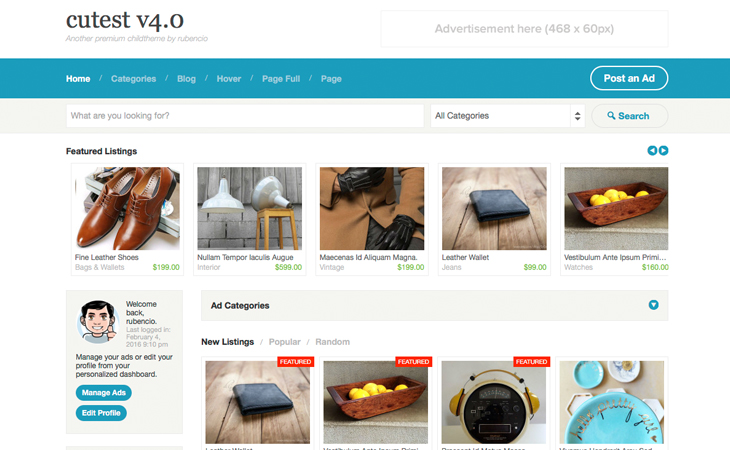In this image, we're examining a website interface prominently displaying the title "Cutest V4.0" at the top left, identifying it as another premium child theme by Rubindo. On the top right corner, there's an advertisement banner labeled "468x60PX," set against a blue background.

The navigation bar spans from left to right, featuring various categories: "Home" (highlighted in white) followed by "Categories," "Blog," "Hover," "Pageful," and "Page" in gray text. Positioned to the right is a white oval button with the text "Post an Ad".

Below the navigation bar, there's a search section prompt, "What are you looking for?" alongside a dropdown menu labeled "All Categories," and a search button.

The main content area showcases featured listings with five different images. Green price tags accompany diverse products titled "Five Leather Shoes," "Newland Temper," "Turriculous Ag," a non-English description, "Leather Wallet," and a basket of yellow fruit.

Towards the bottom left, there is a personalized welcome message: "Welcome Back, Rubinco," followed by options to manage ads or edit the profile via two blue buttons labeled "Manage Ads" and "Edit Profile".

On the bottom right, the site contains three categories: "New Listings," "Popular," and "Random," each accompanied by four square images of items available for sale.